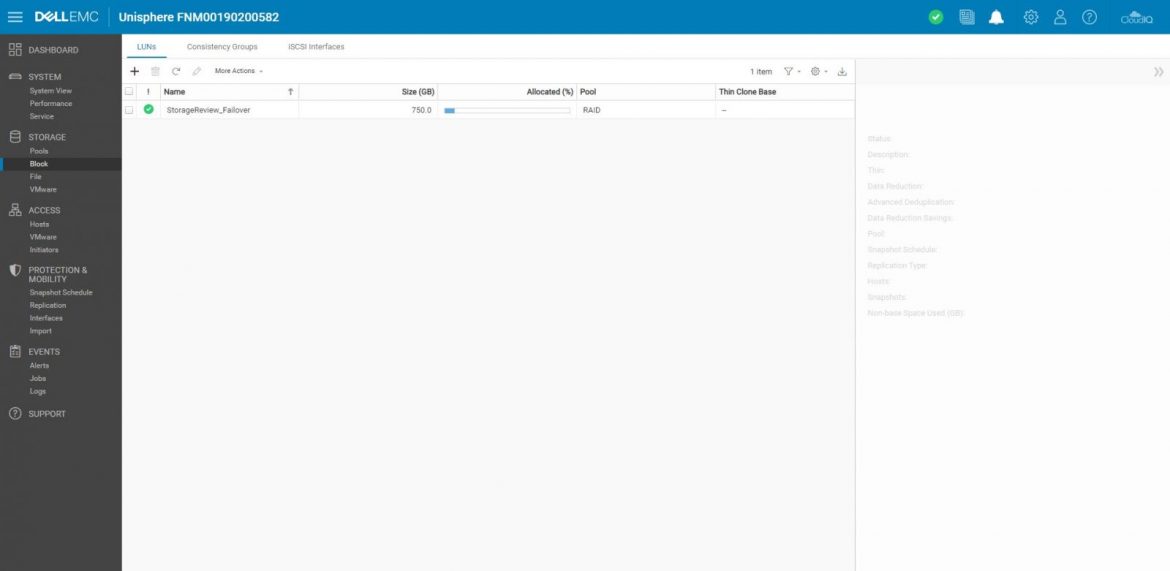This screenshot captures the interface of Dell EMC Unisphere, a storage management system. At the top of the screen, a blue bar displays the title "Dell EMC Unisphere" followed by numerical identifiers. Towards the right section of this bar, there are several icons, including a green circle with a check mark indicating system status.

On the left side, a vertical black bar is present, housing a navigation menu. Key menu items such as "Dashboard," "System," and "Storage" are listed, with "Block" selected under "Storage."

The central portion of the screen features a grayish rectangle, where an underlined blue link labeled "LUNS" is prominent. This area appears to display details such as "Name," "Size," "Allocated Percentage," "Pool," "Thin Close," and "Base." Additionally, a green circle with a check mark is visible beside the word "Storage Review." Below this, a progress bar with a small section filled in blue shows usage percentages.

The overall layout of the screen is minimalistic, with significant white space surrounding the interface elements.